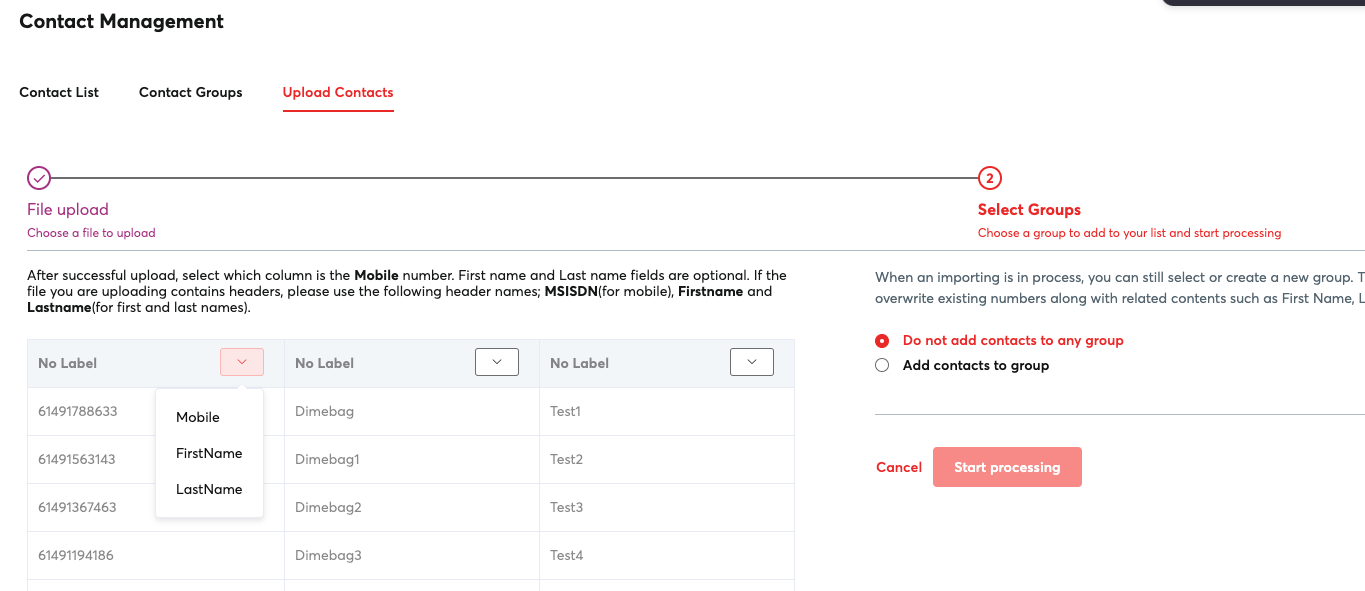A detailed descriptive caption for the image could be:

"This screenshot depicts a contact management form interface. At the top left corner, the title 'Contact Management' is prominently displayed. Directly beneath the title, there are three navigational tabs labeled 'Contact Lists,' 'Contact Groups,' and 'Upload Contacts,' with the 'Upload Contacts' tab highlighted in red. Further below, a purple checkmark is illustrated, linked via a black line to a red numeral '2'. To the right of this visual icon, the section titled 'File Upload' is found under the checkmark, prompting users to select and upload a file. Adjacent to this on the right side, there's another section titled 'Select Groups,' which guides users to choose a group for adding contacts and initiating the process. Below these sections, a table appears with three columns, each labeled as 'No Label,' and featuring a drop-down icon. To the far right, two sets of radio buttons are visible, one labeled 'Do Not Add Context' and the other 'Group and Add Context.'"